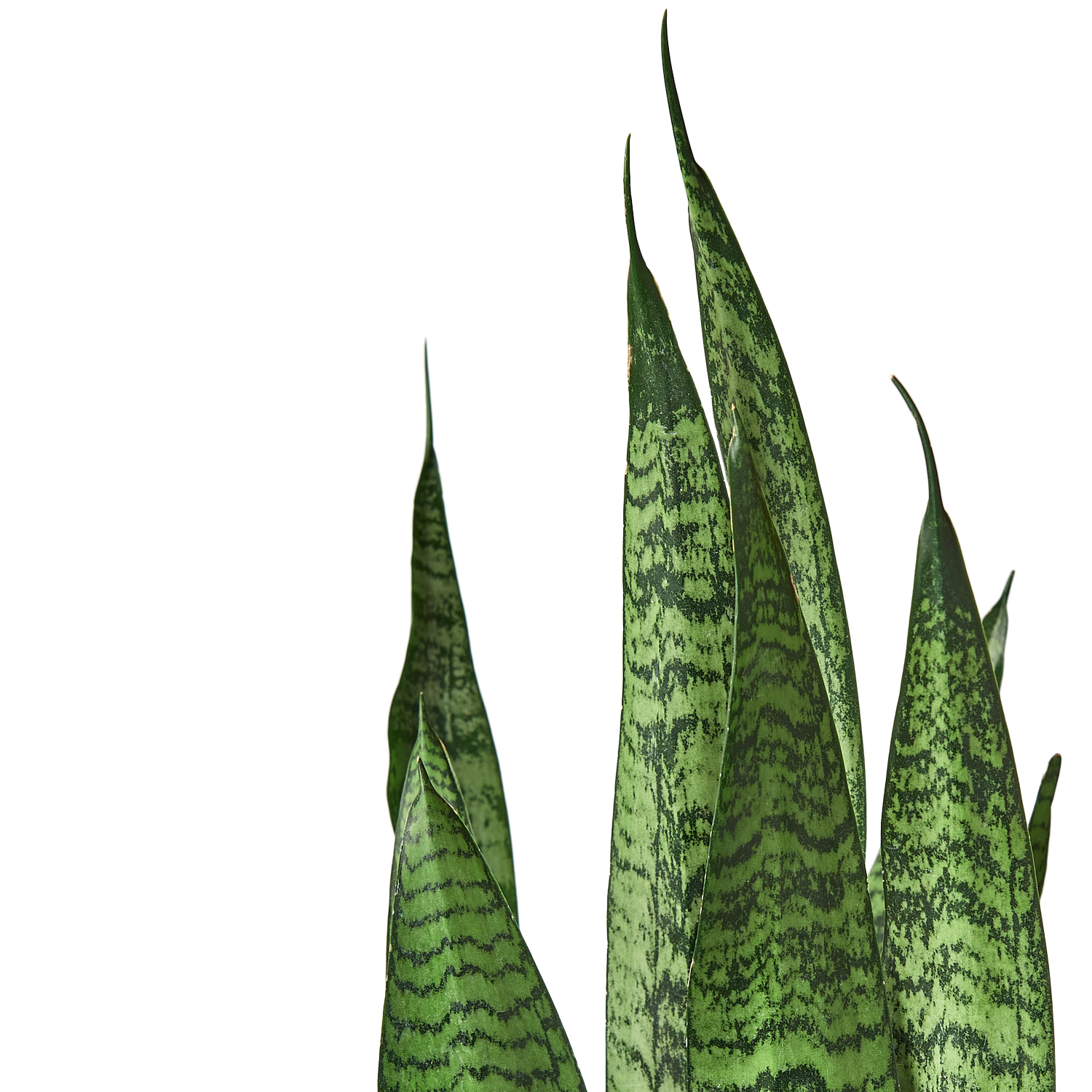The image depicts the upper part of a Sansevieria plant, commonly known as mother-in-law's tongue or snake plant, set against a white background. The photograph focuses solely on the tips of nine spear-like leaves, which are sharply pointed and become narrower towards the top. These leaves exhibit a striking pattern of light green to dark green hues, interspersed with darker green spots or irregular horizontal stripes. The tallest leaf is positioned in the center, with the remaining leaves gradually becoming shorter, all appearing robust and healthy. The bottom portion of the plant, including the pot or roots, is not visible in the picture, highlighting only the elegantly variegated and pointed foliage.